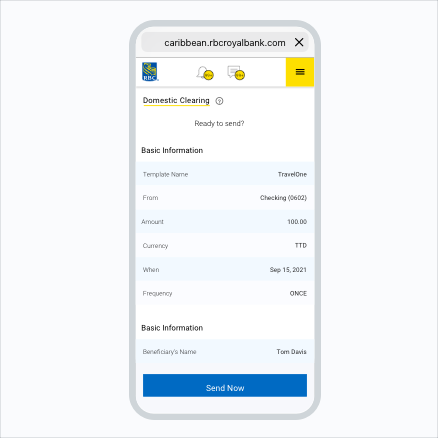The image displays a mock-up of a smartphone with a banking app open, specifically the Caribbean branch of RBC Royal Bank, as indicated by the URL caribbean.rbcroyalbank.com. Dominating the top-left corner is RBC's signature SHIELD logo. The interface on the screen is quite small and difficult to read, showcasing a bank transaction in progress. At the top of the screen, the header reads "Domestic Clearing, ready to send."

The transaction details are as follows:
- **Template Name**: Travel One
- **From**: Checking account "indian0602"
- **Amount**: 100 (currency unclear, potentially USD or GBP)
- **When**: September 15, 2021
- **Frequency**: Once

Further down the screen, additional transaction details are visible, including the beneficiary's name, "Tom Davis." The content appears to continue beyond this point, but the page display cuts off here. At the bottom of the screen is a prominent blue "Send Now" button, ready for the user to confirm the transaction. Overall, the image captures a moment where someone is preparing to send money through their mobile banking app.